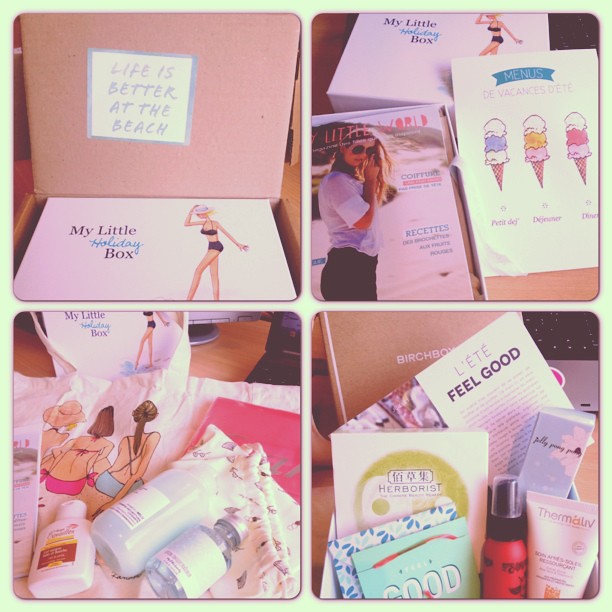This image is a square-shaped collage with a neon-green background, displaying four separate photos arranged in a grid with rounded corners and white divider lines. The upper left photo features a pink box with its lid open, revealing the message "Life is Better at the Beach" in a square white panel with a purple border. Inside the box, another package labeled "My Little Holiday Box" depicts a woman in a black bikini and white hat. The upper right photo shows the same "My Little Holiday Box" but also includes a women's magazine titled "Little World," featuring a photo of a woman. Below this, a card displays three ice cream cones with a blue banner reading "Menus" and possibly text in a foreign language. The cones are colored white, blue, white; red, yellow, white; and pink, red, white. The lower left photo captures the contents of "My Little Holiday Box" again, along with beach-themed clothing, bottles of suntan lotion, and other skincare products on a white table. The bottom right photo exhibits a gift basket containing additional boxes, books, greeting cards, and a variety of cosmetic products, which could include make-up primers and lotions.